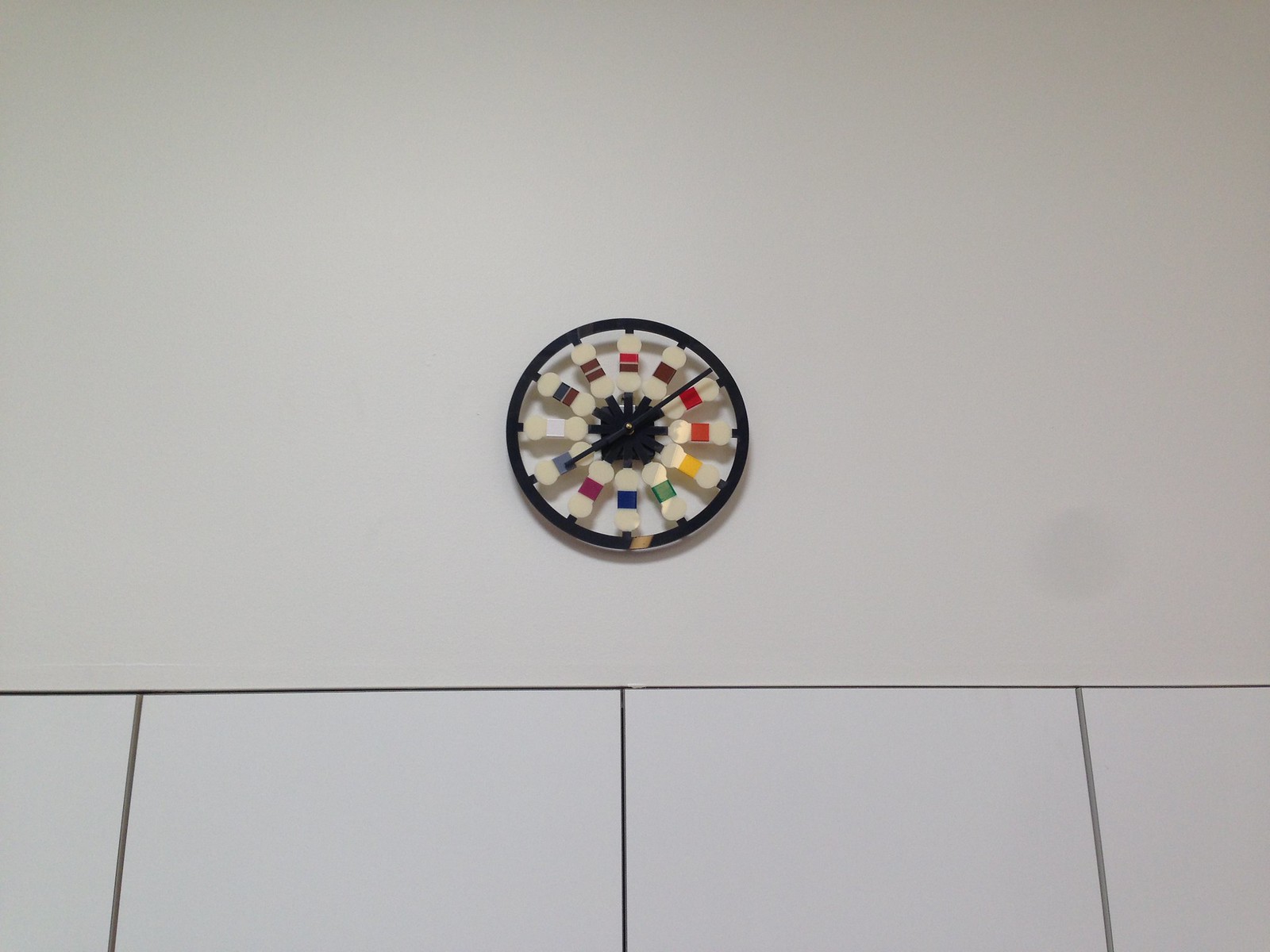This color photograph, taken indoors, prominently features an off-white wall with a distinctive wall clock centered in the image, occupying approximately 15-20% of the frame. The clock has a black bezel and a single visible black hand, the other hand being directly behind it, secured by a silver button at the center. Unusually, instead of numbers, the clock face displays various snowboard-shaped segments adorned with colorful stripes: pink and brown at twelve, brown at one, blue at six, purple at seven, along with red, yellow, green, maroon, gray, and white in other positions. Below the clock, four large white panels—possibly tiles or closet doors—span the lower portion of the wall, divided by noticeable lines, adding a structured, segmented look to the scene.